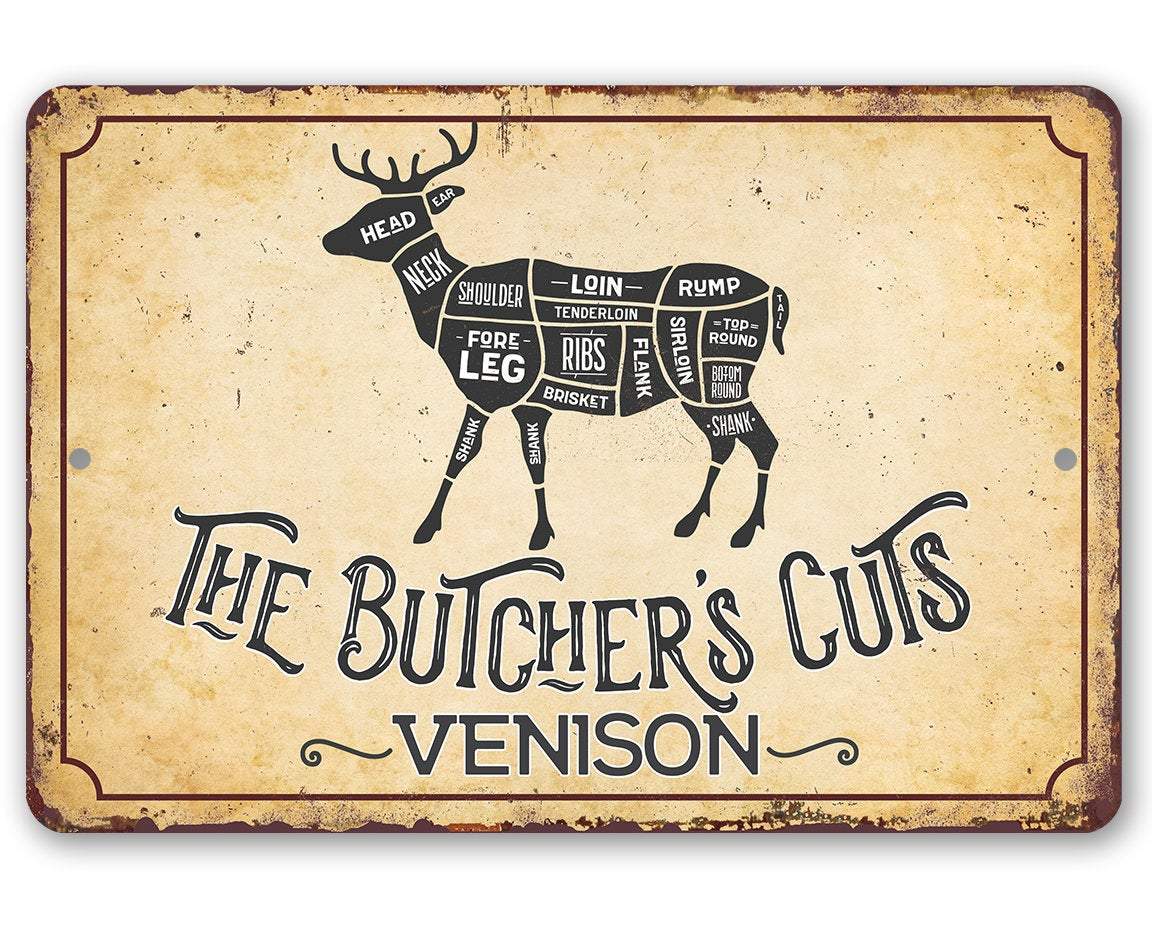The image is an antique-looking butcher guide for venison, presented on a rectangular background with rounded edges that shows signs of wear with a beige color and faded red along the border. Inside this, there is a thin, red outline with inverted, curved corners. Dominating the center-top of the frame is a silhouetted image of a deer with all its parts meticulously labeled in white text: head, ear, neck, shoulder, foreleg, shank, shank, loin, tenderloin, ribs, brisket, flank, rump, sirloin, top round, bottom round, and tail. Below the deer, elegant black text with a white interior spells out "The Butcher's Cuts," followed by the word "Venison" in bold black text outlined in white, flanked by ornate black curls. This detailed depiction effectively demonstrates how a deer is segmented into various cuts of meat, offering a clear and educational view of the process.